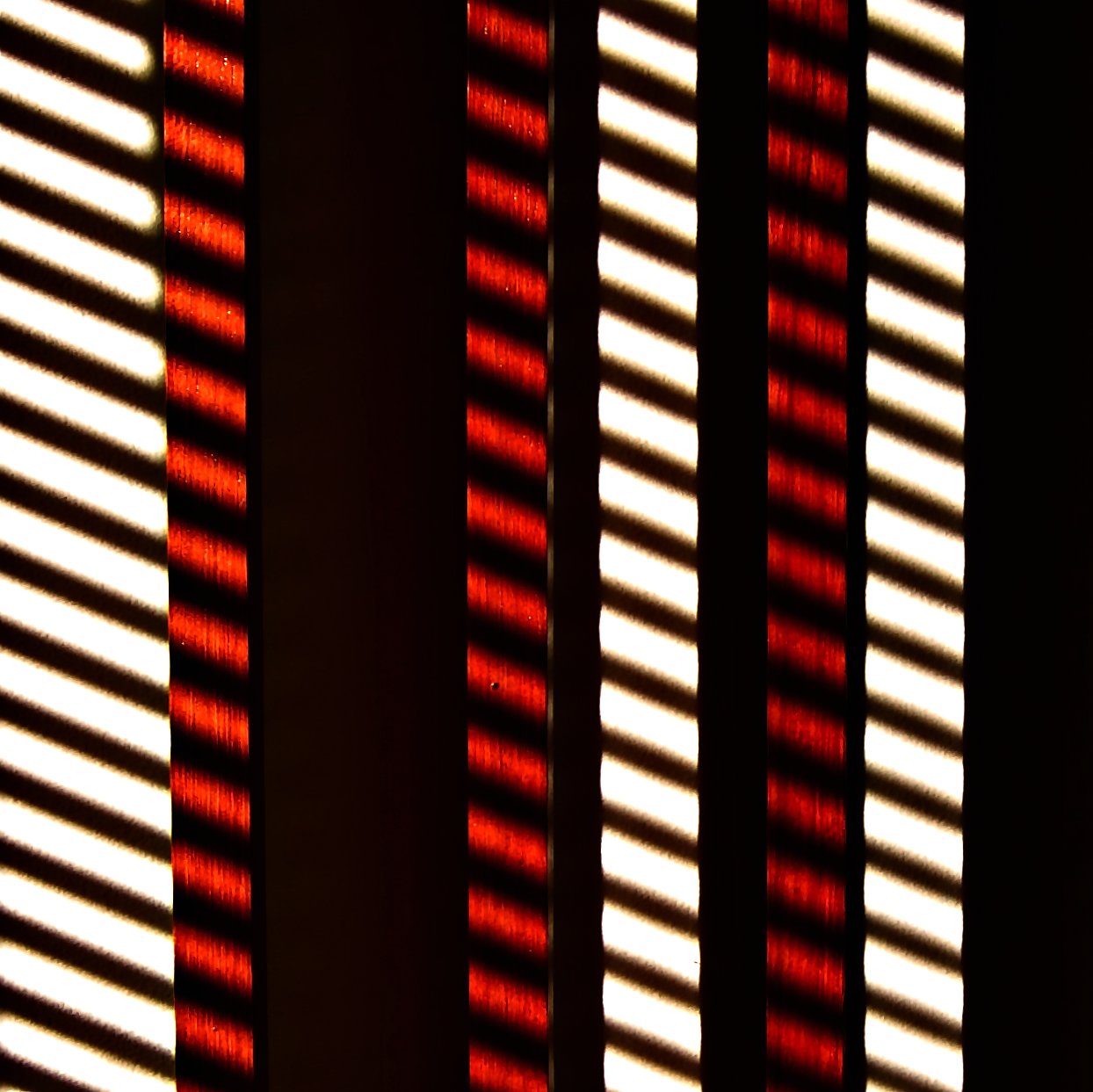This abstract image features a series of white and red stripes arranged in several strips across a predominantly black background. The overall design is centralized but slightly offset to the left. The pattern includes rows of white and red elements that resemble lights. The white lights are more elongated and rectangular, while the red lights are smaller and thinner. The arrangement is evenly spaced, creating a repetitive sequence of white lights, red lights, and dark spaces. Notably, there is a small circular dot positioned centrally within the design. The image lacks any discernible text or clear indications of what the objects represent, giving it a futuristic or indeterminate aesthetic.